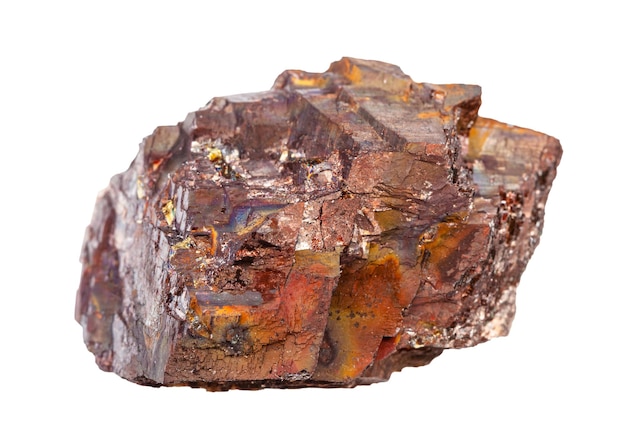This image is a highly detailed, photorealistic close-up of an unpolished mineral displayed against a blank white background. The mineral exhibits multiple jagged and angular edges, contributing to its rough and raw appearance. Its predominant color is a mottled brown, accompanied by sections of white, rust, yellow, olive green, and hints of orangey-red hues. There are also subtle metallic speckles that reflect a rainbowish sheen, potentially indicating traces of various minerals or crystalline structures within the rock. The light source is positioned on the left side, accentuating the flat planes and fractures of the mineral with a reflective highlight, while the front and upper edges remain irregular and jagged. Despite its varied colors and textures, there are no labels or text identifying the specific type of mineral, leaving it open to interpretation.